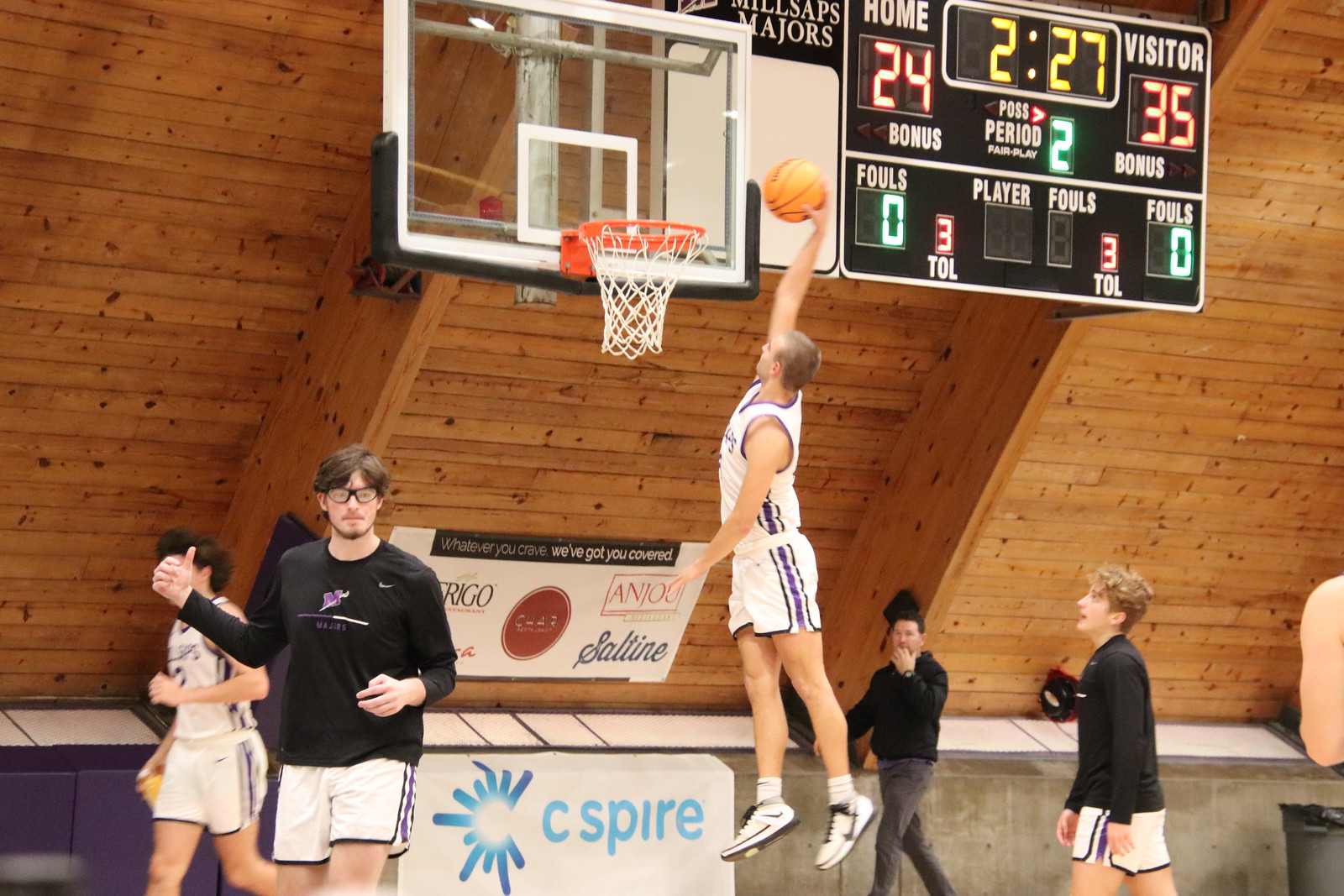The image captures an intense moment in an indoor gymnasium as a basketball player in mid-air prepares to dunk a ball into the hoop. The player, dressed in a white uniform with blue stripes down the sides of his sleeveless jersey and shorts, and white shoes, is poised with his arm extended towards the basket while his other arm is down. The player's left side faces the camera, showcasing the determined expression on his face. The basketball hoop is mounted on a large, curved wooden spine attached to a sloping wooden wall, which adds a unique architectural element to the background. Above the hoop, a digital scoreboard displays the score with 2 minutes and 27 seconds remaining, showing the visitors leading the home team 35-24, and no fouls on either side. Various onlookers and individuals in similar jerseys and black shirts, including one giving a thumbs up, surround the player, highlighting the intensity and anticipation of the moment. The pristine, wooden ceiling of the gymnasium extends overhead, contributing to the clean, well-maintained atmosphere of the setting.